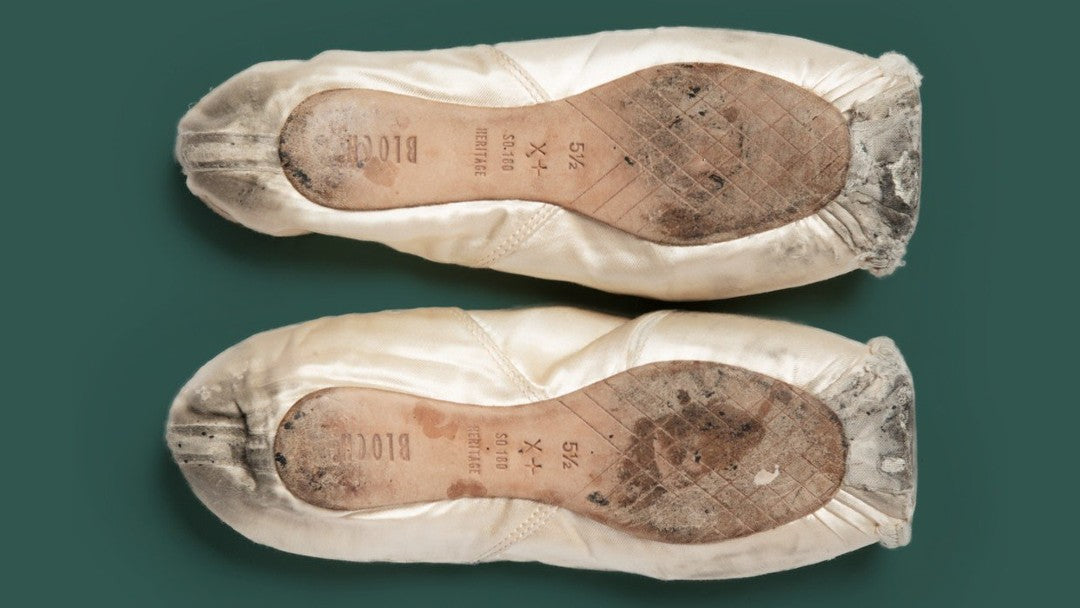The image features a pair of worn-out ballet shoes positioned upside down on a dark green surface. The ballet shoes have a white body with peach-colored soles that reveal significant wear, evident through the flattened and damaged toe areas and numerous black skid marks. The soles, likely made of a beige rubber, display a size marking of "five and a half" along with additional codes like "SO180 heritage." Despite their elegant design, with satin or silk-like material on the borders, the shoes exhibit considerable dirt and grime, especially on the heels and the underside.